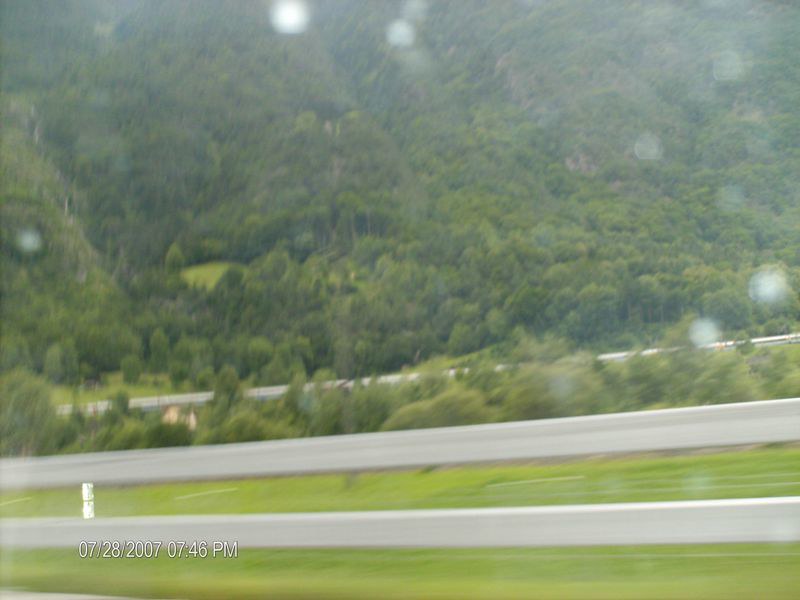This photograph captures a serene nature landscape, likely taken from within a moving vehicle, as suggested by the evident glare and motion blur. The scene features a sprawling green pasture, bathed in daylight, leading to a distant hill densely populated with towering trees. The grass exhibits a light yellowish-green hue, contrasting with the more vibrant and lush green of the trees, which resemble the texture of cauliflower. The distant perspective makes these sizable trees appear deceptively small. The timestamp in the bottom left corner of the image indicates it was taken on July 28, 2007, at 7:46 p.m., evidencing its origins as a digital photo.